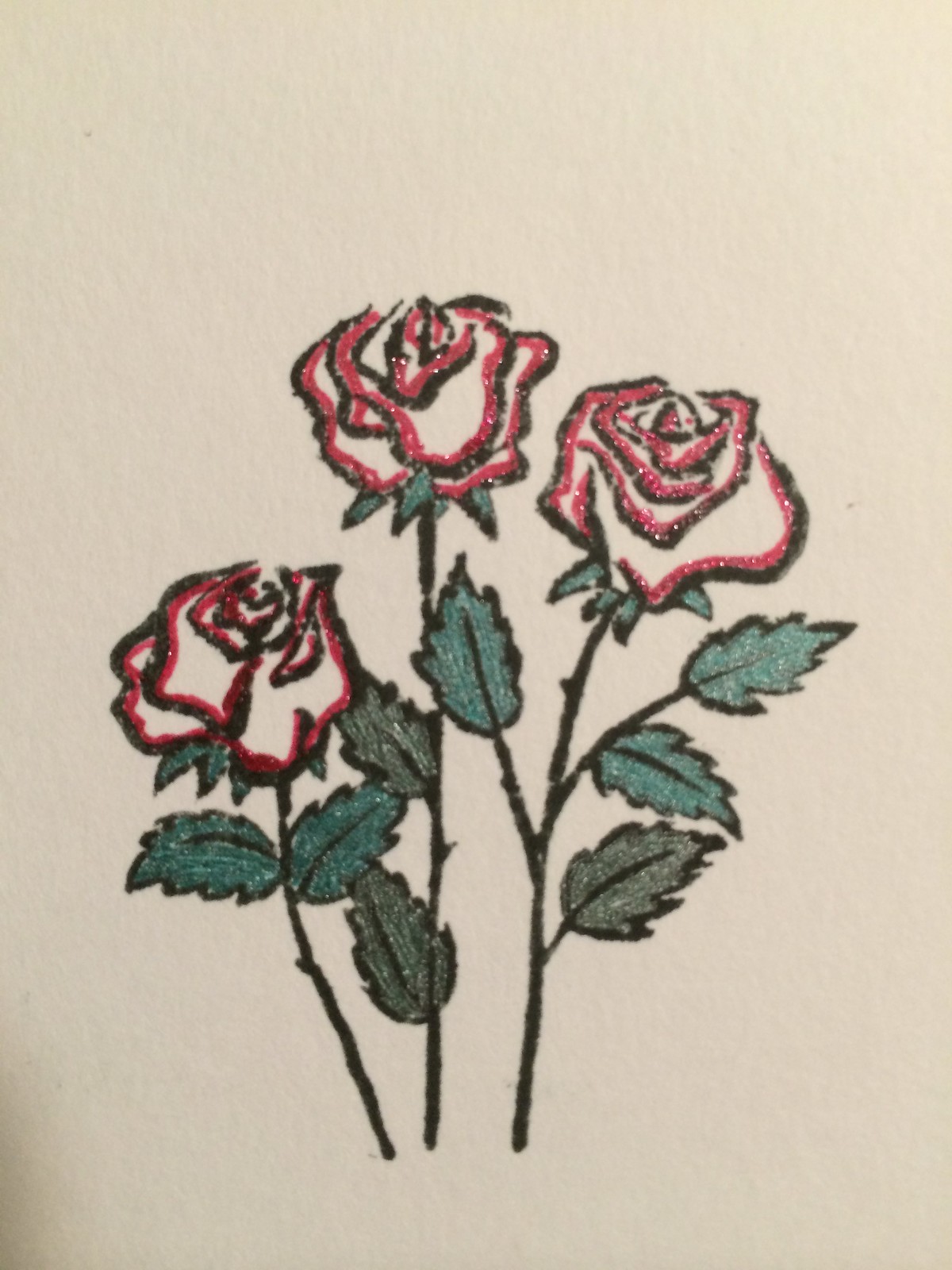This image showcases a detailed ink drawing of three roses on off-white, light tan, cream-colored paper. Centrally placed, the roses vary in height: the first is the shortest, the middle one is the tallest, and the third is slightly shorter than the tallest. The roses feature intricate dual outlines, combining black ink with adjacent red markers, lending a striking, colorful contrast. The petals themselves remain uncolored, allowing the paper's natural hue to show through. Enhancing the roses' borders, a layer of sparkly silver glitter adds a touch of shimmer.

The roses are supported by straight, thick stems, illustrated in black or dark green ink, some embellished with tiny thorns. Each rose is adorned with jagged-edged leaves, presenting a black outline and central vein. The leaves are filled in with shades of green, varying from light to dark, with a possible glitter overlay for added effect.

The first rose features two leaves—one on each side—with additional green beneath the top part of the rose. The middle rose has two darker green leaves on one side, complementing the bloom. The third rose displays a combination of both lighter and darker green foliage, with one leaf on the left and three on the right, underlining the illustrated roses' intricate detail and layered coloration.